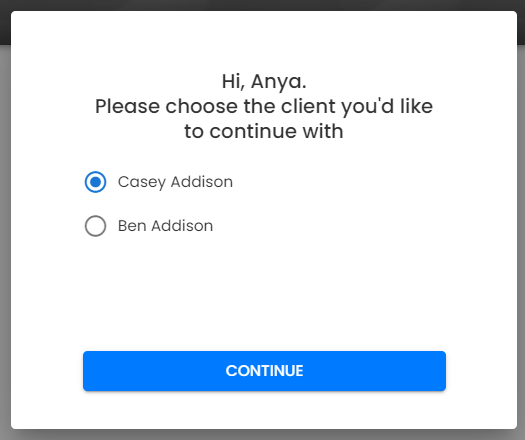In the center of the image, there is a prominent white dialogue box with a message that reads, "Hi Anya, please choose the client you'd like to continue with." The interface is framed by gray edges. Below the message, there are two options presented in blue rectangles: one for Casey Addison, labeled as 'checked' to indicate it is selected, and one for Ben Addison, labeled as 'not checked.' The blue rectangles are clearly defined against the white backdrop of the window. The entire composition is organized in a clean, straightforward manner, emphasizing the importance of the user selection process.